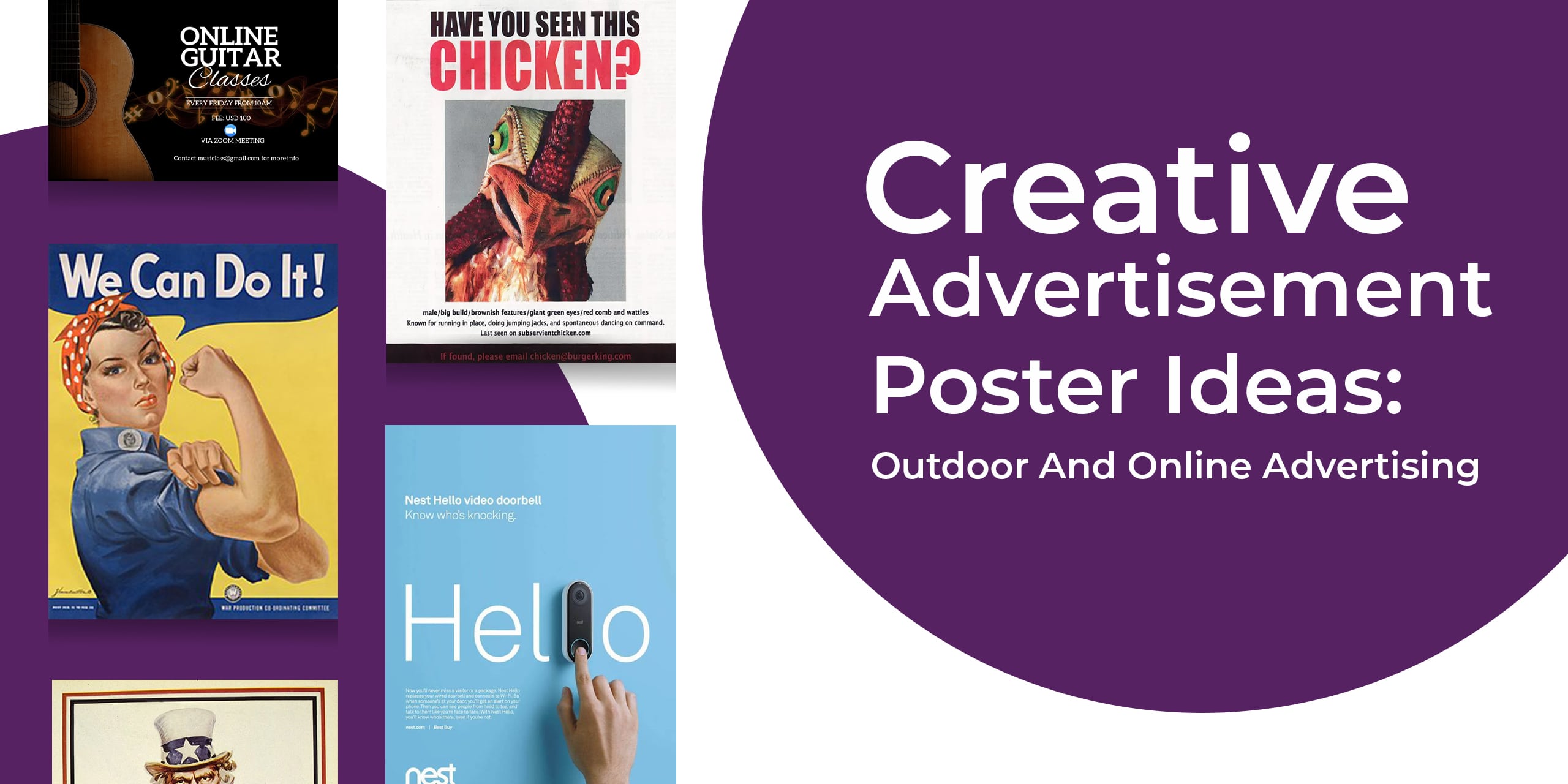This advertisement, designed in a landscape layout, is split into two sections: a right and a left half. The right half features a semi-circle in a deep purple color, partially cut off at the corner, containing white text that reads, "Creative Advertisement Poster Ideas: Outdoor and Online Advertising." The left half showcases a collection of five different posters. The topmost poster stands out with its black background and an image of a guitar, promoting "Online Guitar Classes." Directly below this is the iconic Rosie the Riveter poster, displaying the determined figure with her red and white handkerchief, flexing her muscle, and the empowering slogan, "We Can Do It." Further down, partially cut off, is the famous Uncle Sam poster with his distinctive white hat decorated with blue stars. To the right, a quirky advertisement features an image of a chicken under the headline, "Have You Seen This Chicken?" At the bottom, a blue rectangle highlights the Nest alarm system, featuring the Nest logo, a device resembling a doorbell, and the word "Hello." The diverse collection of posters serves as a creative example of both outdoor and online advertising techniques.